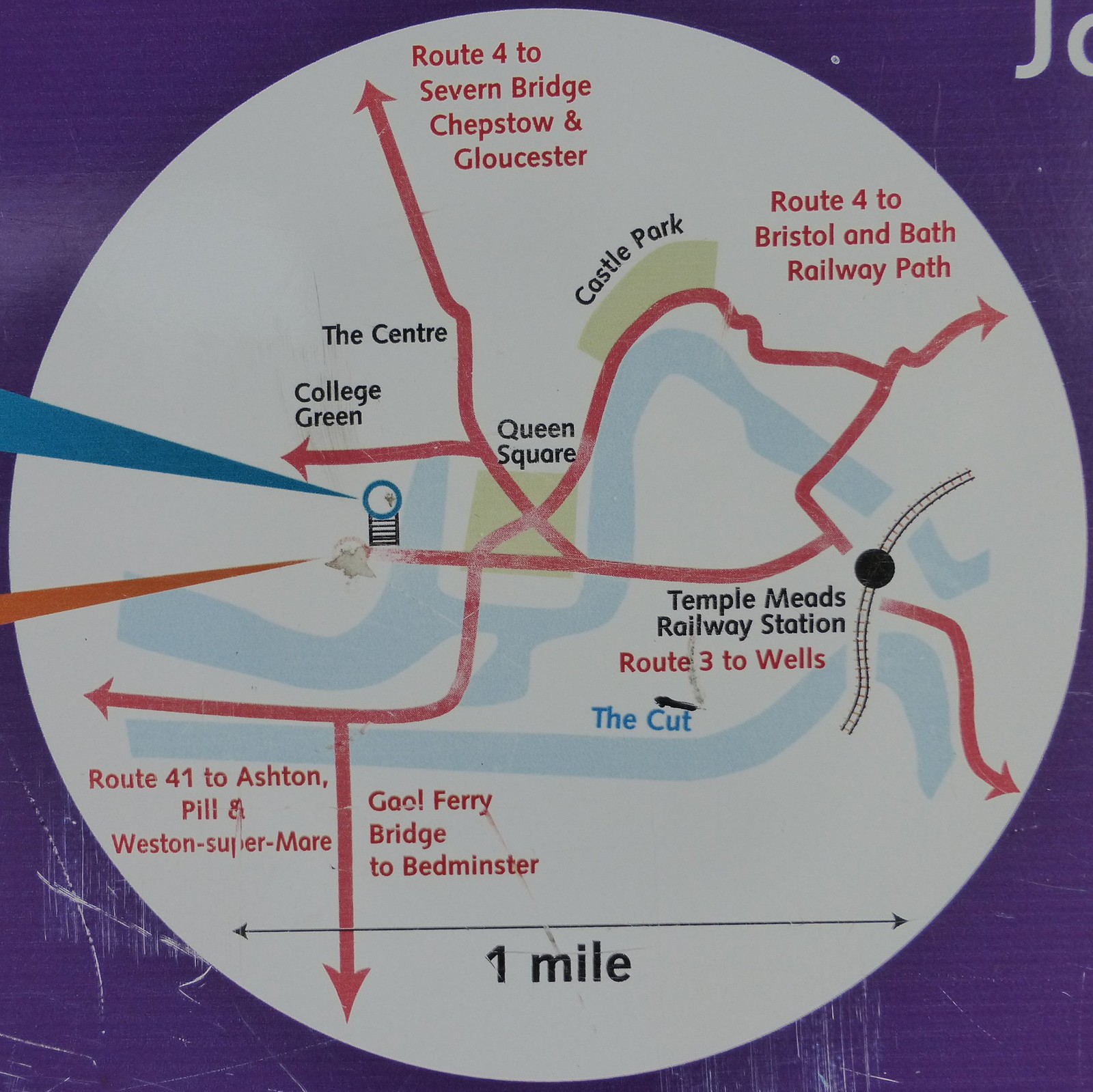This image features a detailed map encased within a round grayish-white circle, prominently positioned against a scratched purple background. The circular map reveals various routes marked in red lines, interspersed with parks, rivers, and railroads. At the top, bold red text states "Route 4 to Severn Bridge, Chepstow, and Gloucester." Inside the circle, key locations are denoted: the Center, College Green near the top middle, Queen Square at the center, Castle Park to the left, Temple Meads Railway Station to the right, and The Cut. Routes extend outward, including Route 4 to Bristol and Bath Railway Path at the upper right, Route 3 to Wells, and Route 41 to Ashton, Pill, and Weston-Super-Mare on the bottom left. Additionally, Gould Ferry Bridge to Bedminster is marked next to Route 41. At the bottom, a scale indicates a distance of one mile. The entire map is marked by numerous white scratches, especially noticeable towards the bottom.